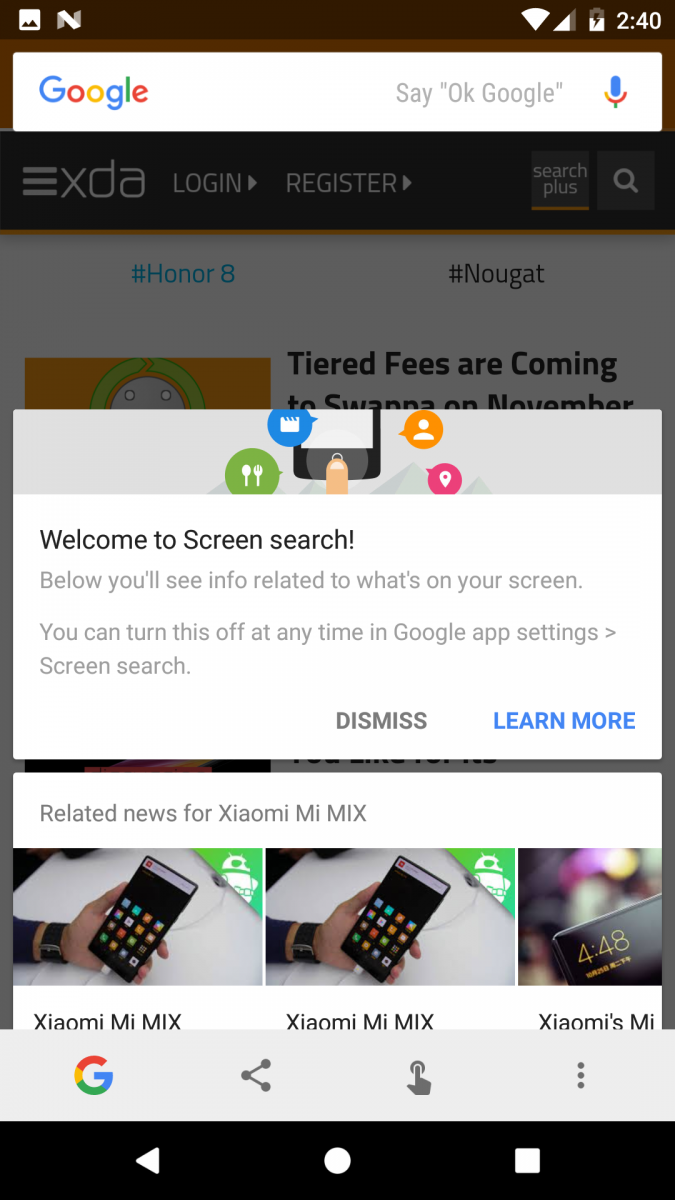A detailed screenshot of a phone screen displaying Google search features. The time on the phone is 2:40. At the top, there's a search bar open to Google, with the iconic Google logo on the left, showcasing its usual colors: blue, red, yellow, blue, green, and red. A microphone icon next to the search bar invites users to "Say 'OK Google'" for voice search.

Below the search bar, there's a section with icons for a hamburger menu and "XDA," possibly referring to XDA Developers, a popular mobile software development community. It provides options to log in or register.

Further down, several terms are displayed, including "Honor" and "Nougat." A logo appears beside text about "tiered fees are coming," followed by what looks like a Siri logo. 

A gray text box welcomes the user to screen search and explains that it shows information related to what's on the screen, with an option to turn off the feature in the Google app settings. Below this information, there are buttons in gray and blue that allow the user to "Dismiss" or "Learn more" about the screen search feature.

Finally, there's a section titled "Related news for Zenomi My Mix," which could refer to a phone or a calculator. Several clickable options are available to explore new features or updates related to this topic.